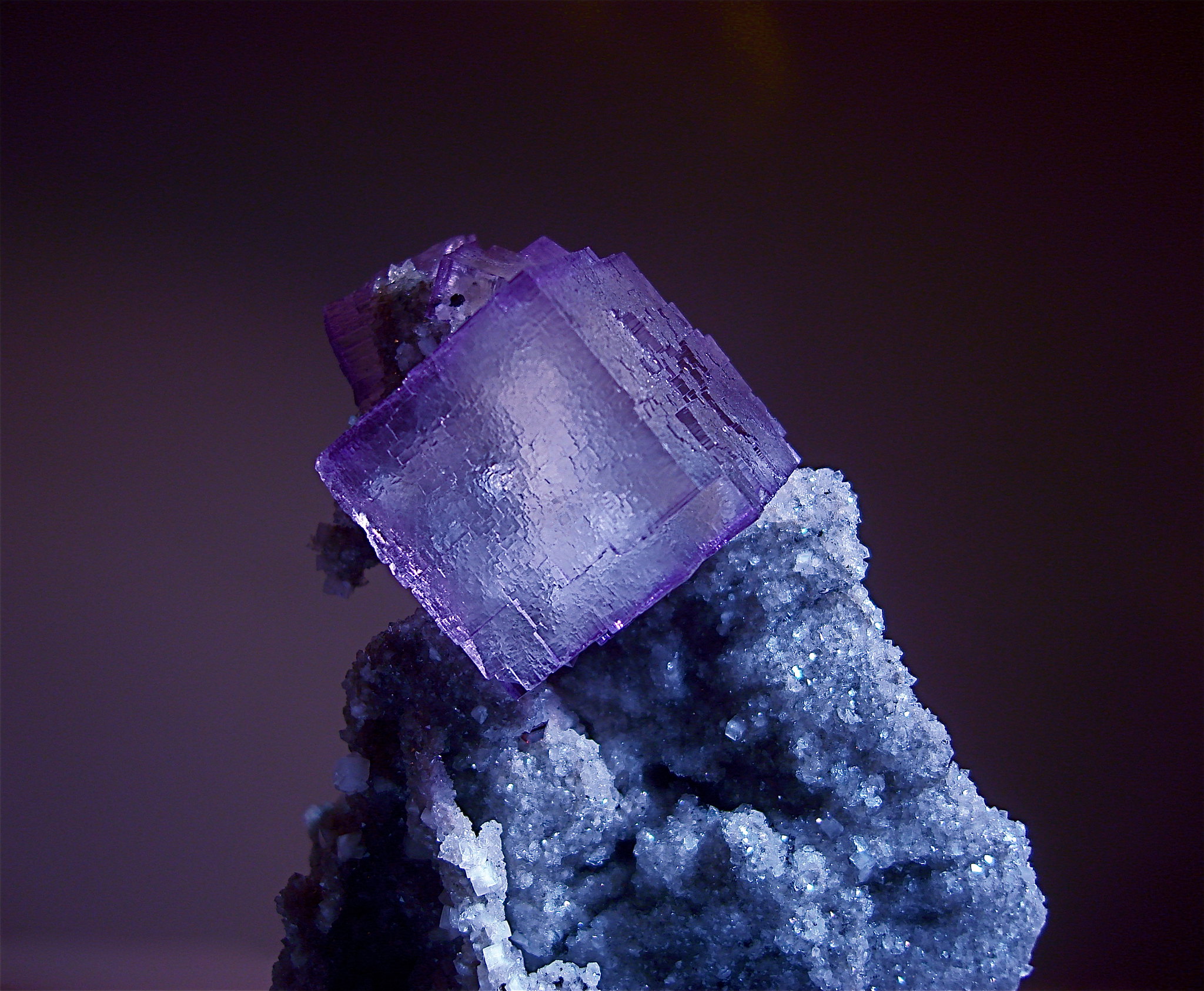A detailed caption for this image could be:

"In this captivating photograph, a mesmerizing crystallized geode takes center stage. The geode features an intriguing formation, where a perfectly square, dark purple crystal is perched at an angle leaning to the left. The geode's base intriguingly mimics the appearance of two fingers and a knuckle, as if gently holding up the square crystal. On the left side, the support resembles a thumb, adding to the lifelike illusion. The square crystal, with its smooth surface, exudes an icy texture, enhanced by its purple hue. The backdrop of the image is an ombre gradient of purple, transitioning from dark at the top to light in the center, and fading back to dark again in the bottom right corner. The lighter purple of the geode’s crystallized formations contrasts beautifully with the deeper purple of the embedded square crystal."